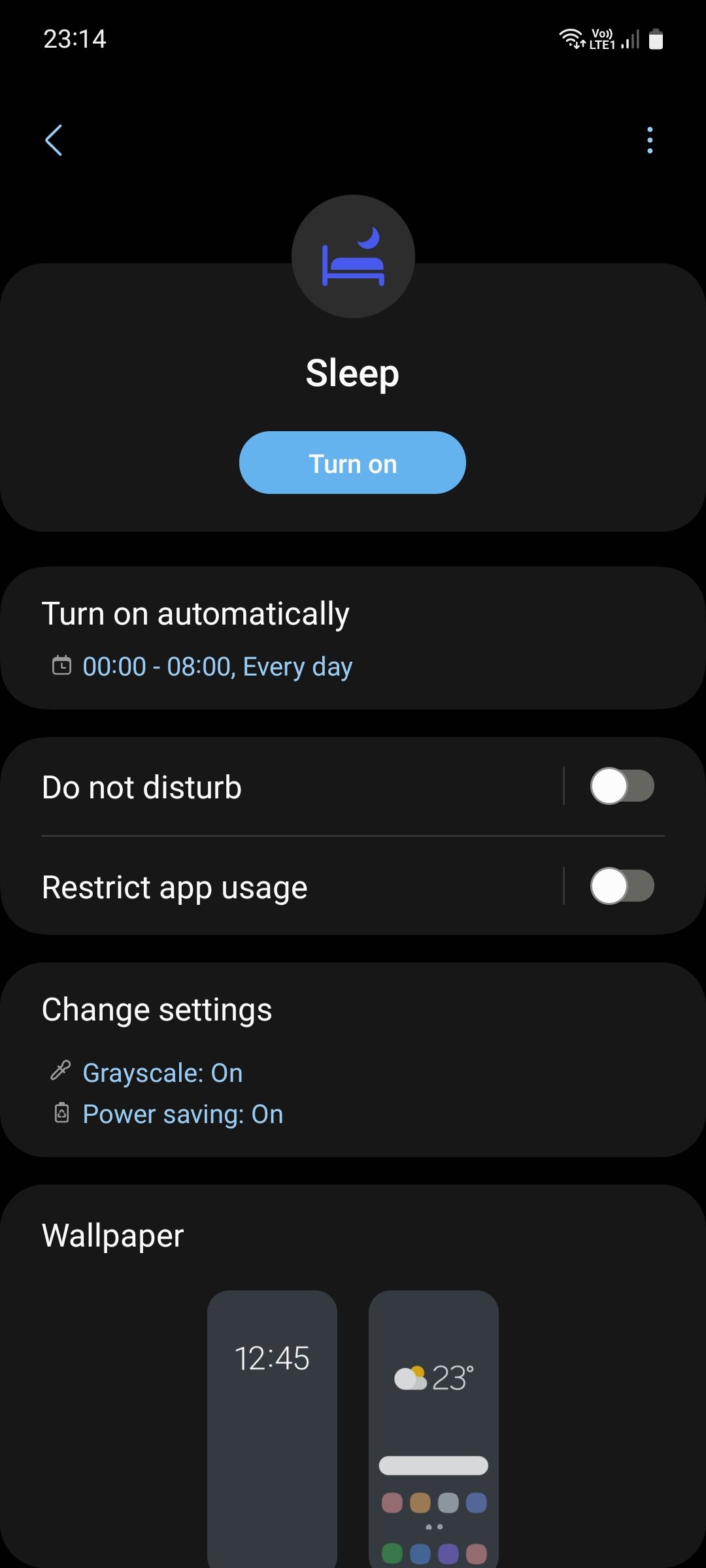The image depicts a smartphone screen with various settings and notifications. The screen has a black background and the following details:

1. **Top Left Corner**:
   - The time reads "23:14".

2. **Top Right Corner**:
   - Indicators for mobile data, Wi-Fi signal strength, cellular signal bars, and a full battery icon.

3. **Central Section**:
   - An arrow icon on the left and a three-dot menu icon on the right just below the status bar.
   - The word "Sleep" is prominently displayed in the middle.
   - A blue button with white text that reads "Turn On".
   - Beneath the button, the text "Turn on automatically 00:00 through 08:00 every day" is visible.

4. **Settings Area**:
   - A toggle switch for "Do Not Disturb," which is turned off.
   - A toggle switch for "Restricted App Usage," which is also turned off.
   - Options for setting: "Change Settings" for grayscale, "Power Saving" mode, and "Wallpaper."
   - The wallpaper option shows an entry labeled "1245."

5. **Wallpaper Description**:
   - A simple black wallpaper.
   - Another wallpaper featuring weather information with a cloud and sun icon, indicating 23 degrees.

6. **Apps and Colors**:
   - A bar with icons representing various apps displayed as different colors.
   - The colors include various shades of blue, as well as gray, pink, orange, green, and purple.

The overall theme seems to revolve around sleep settings and power management, providing a detailed and organized view for the user.